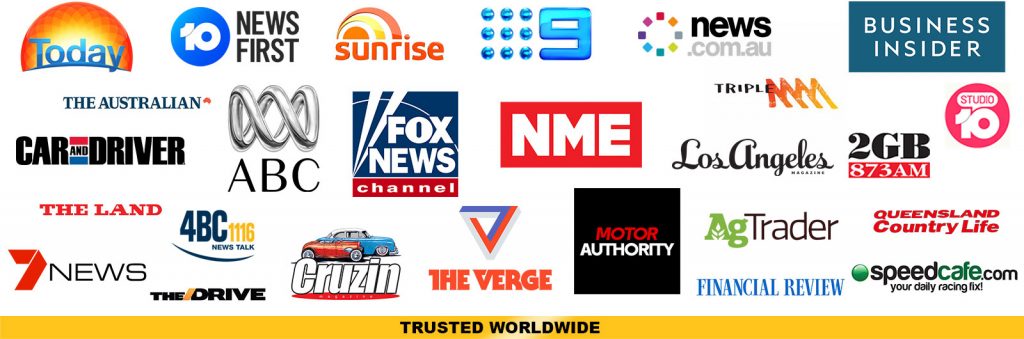This image is a screenshot featuring an array of logos from various TV programs and news outlets, organized in three rows. Each logo is distinct and colorful, reflecting the branding of each respective program or outlet.

### Top Row:
1. **Today**: A blue logo with the word "Today" accompanied by a sunburst graphic.
2. **News First**: A design with a blue circle containing the number "10" in white, and the words "News First" in black alongside it.
3. **Sunrise**: Features the word "Sunrise" in orange with a small half sun in orange next to a yellow beam, and another beam above it in red.
4. **Nine News**: Includes nine blue dots next to the number "9", all in blue.
5. **News.com.au**: A circle of multicolored square ‘confetti’ shapes with the word "News" in black and "com.au" in light gray.
6. **Business Insider**: A blue box with "Business Insider" written inside in white.

### Middle Row:
1. **The Australian**: A blue logo with a small red icon.
2. **Car and Driver**: The words "Car" and "Driver" in black, with a red rectangular box above "and" and a blue rectangle below it.
3. **ABC**: A silver metallic figure resembling a figure eight with an extra circle, below which "ABC" is written in black.
4. **Fox News Channel**: A square logo with the top part in blue, featuring the words "Fox News" in white with spotlight bars, and the bottom part in red with "Channel" in white.
5. **NME**: A rectangular red box containing the letters "NME" in white.
6. **Triple M**: The word "Triple" in black followed by “MM” in an orange to yellow gradient.
7. **Los Angeles Magazine**: "Los Angeles" in black cursive, with “Magazine” in black beneath it.
8. **2GB 873 AM**: "2GB" in black with a red bar underneath reading "873 AM".
9. **Studio 10**: A circle logo with a dark pink background, white interior, and the word "Studio" in pink alongside the number "10" in white.

### Bottom Row:
1. **The Land**: A red logo with "The Land" in red.
2. **7 News**: An orange "7" next to the word "News" in black.
3. **4BC News Talk**: "4BC" in blue next to "1116" in yellow, with "News Talk" beneath them and a blue wispy line.
4. **The Drive**: "The" in black, an orange mark, and "Drive" in black.
5. **Cruisin**: An old-fashioned blue and red car above the word "Cruisin" (spelled "C-R-U-Z-I-N") in black, with a red bar underneath containing more text.
6. **The Verge**: "The Verge" in orange, with a triangle above divided into blue, orange, and white sections.
7. **Motor Authority**: A black square with "Motor" in red and "Authority" in white.
8. **Ag Trader**: "Ag" in green and "Trader" in red.
9. **Financial Review**: "Financial Review" in blue.
10. **Queensland Country Life**: "Queensland Country Life" in red.
11. **Speed Cafe**: "Speed" in black, a green dot, and "Cafe" in green, followed by ".com" in black, with the tagline "your daily racing fix" beneath.

### Footer:
A long yellow bar at the bottom with the words "Trusted Worldwide" written in black.